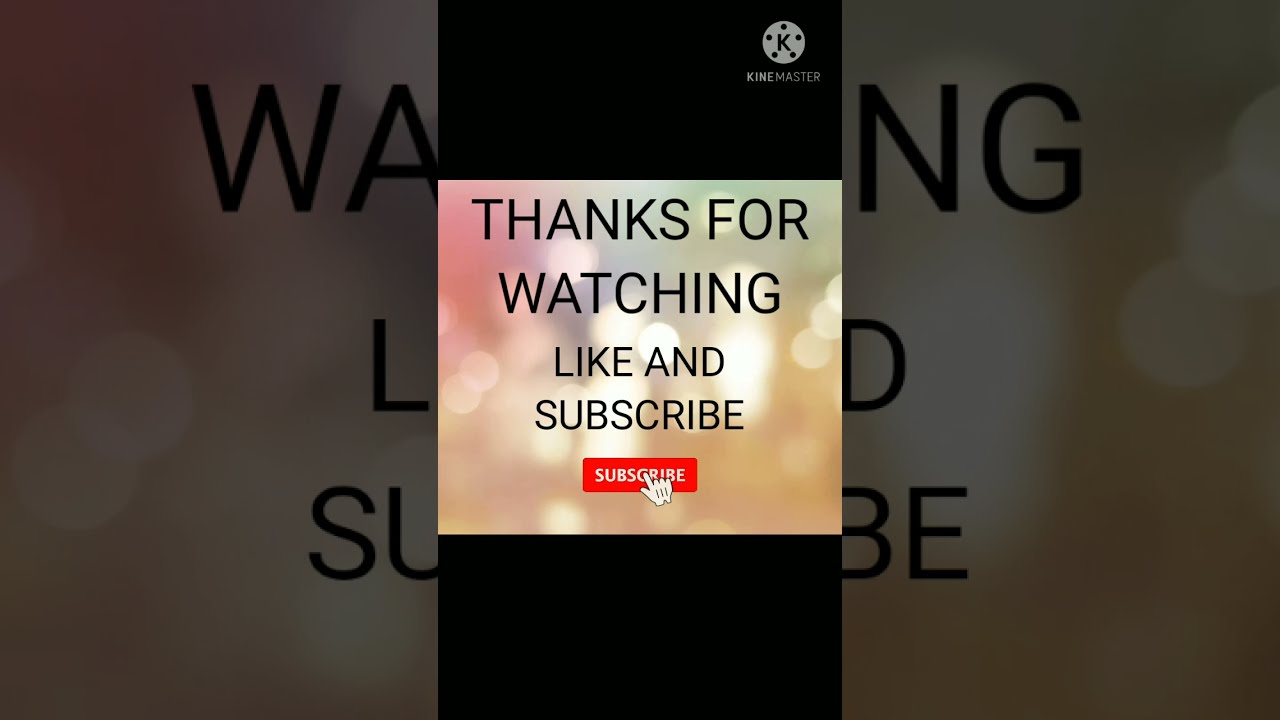The image is a color screenshot from a cell phone displaying the ending screen of a YouTube video, likely using the KineMaster editing app. Central to the image is a message in bold, capitalized black text that reads, "THANKS FOR WATCHING, LIKE AND SUBSCRIBE." Below this text is a red subscribe button with "SUBSCRIBE" in white letters, accompanied by an animated hand icon suggesting to click it. The background features a fuzzy effect of soft, out-of-focus lights in green, blue, white, pink, and yellow hues. On both sides of the central message, the image extends into dark, enlarged sections of the same background design. Black bands are present at the top and bottom of the image. In the upper right corner, the KineMaster logo is visible, consisting of a black "K" within a white circular emblem surrounded by five black dots, with the words "KineMaster" in white on a gray panel below.